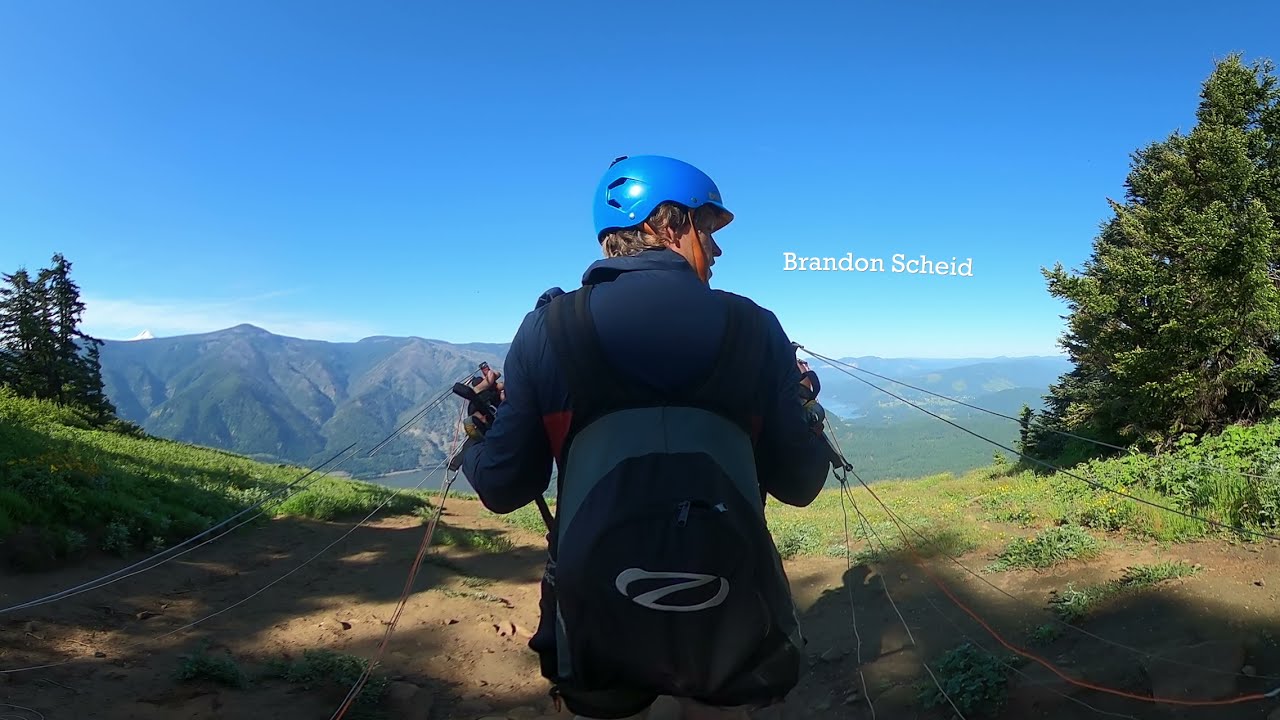The photograph captures the moment before Brandon Scheid embarks on a parasailing adventure. Taken from behind, the image focuses on Brandon, whose name is imposed in white text over the picture. He stands on the edge of a cliff, preparing to leap into the valley below. Brandon is clad in a tall-collared, long-sleeve jacket, and a blue hard hat with an orange chin strap. Black shoulder straps secure a gray and black backpack with a white circular logo on his back. In both hands, he grasps an array of ropes—presumably the lines for his parachute—totaling six in each hand. The backdrop features a light blue sky with scattered clouds, a mix of vegetation and trees flanking both sides, and distant mountain ranges, enhancing the high-elevation setting. The compacted light brown dirt beneath his feet and the precipice in front signal the imminent thrill of his parasailing descent.